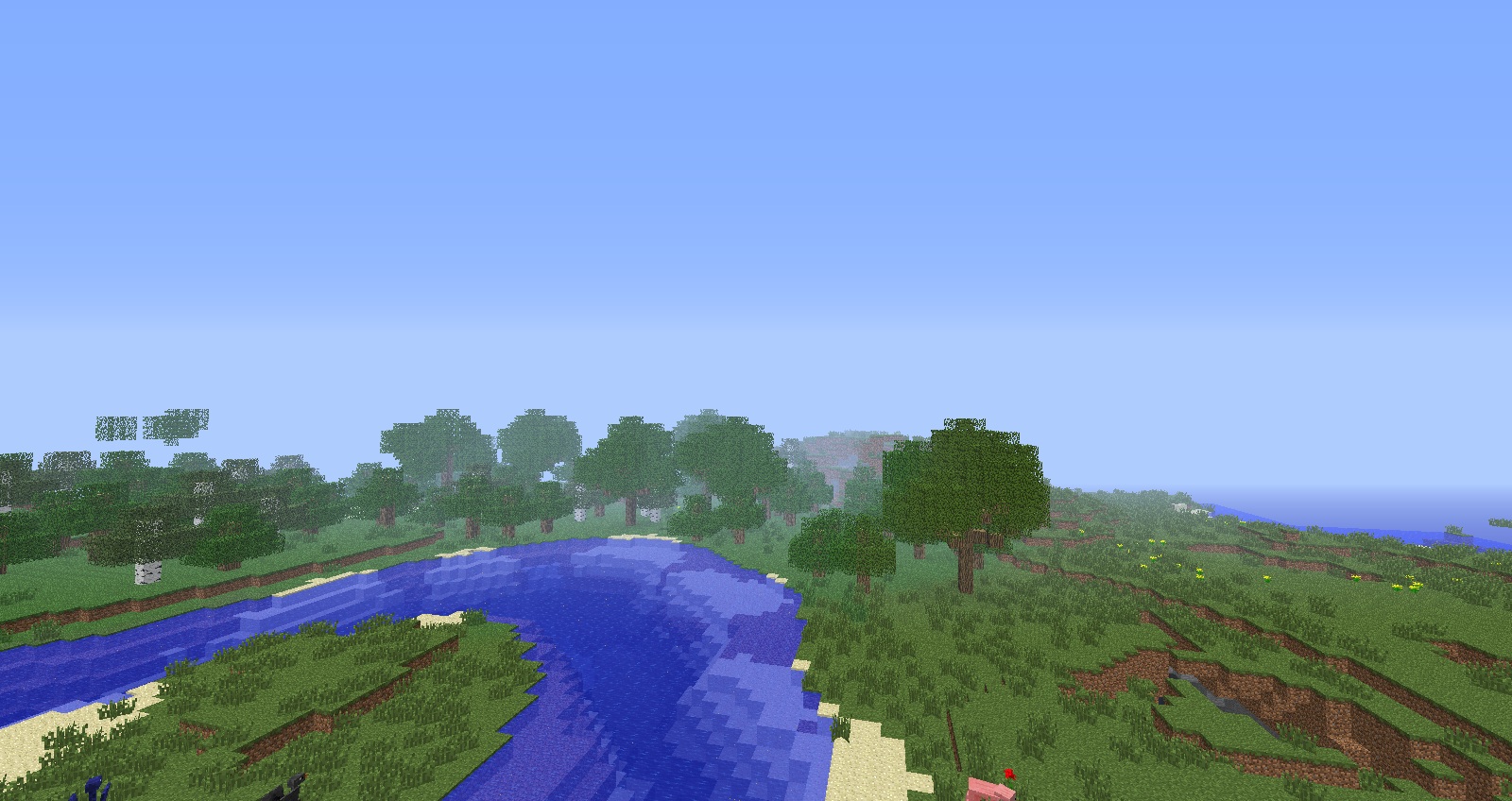This is a rectangular image with the longer side extending horizontally, likely a screenshot from the video game Minecraft. The background predominantly features a clear blue sky with a few hazy clouds concentrated near the bottom edge. Cutting through the scenery is a meandering river that enters from the bottom of the frame, curves upward, and then veers to the left. 

The landscape on both sides of the river is lush and green, peppered with pixelated trees, true to Minecraft's iconic blocky art style. On the mid-right part of the screen, there appears to be an ocean extending into the distance, adding an expansive feel to the scene. The river itself is rendered in tones of blue, accentuated by patches of light tan sand along its banks, enhancing the natural, but stylized, look of the terrain.